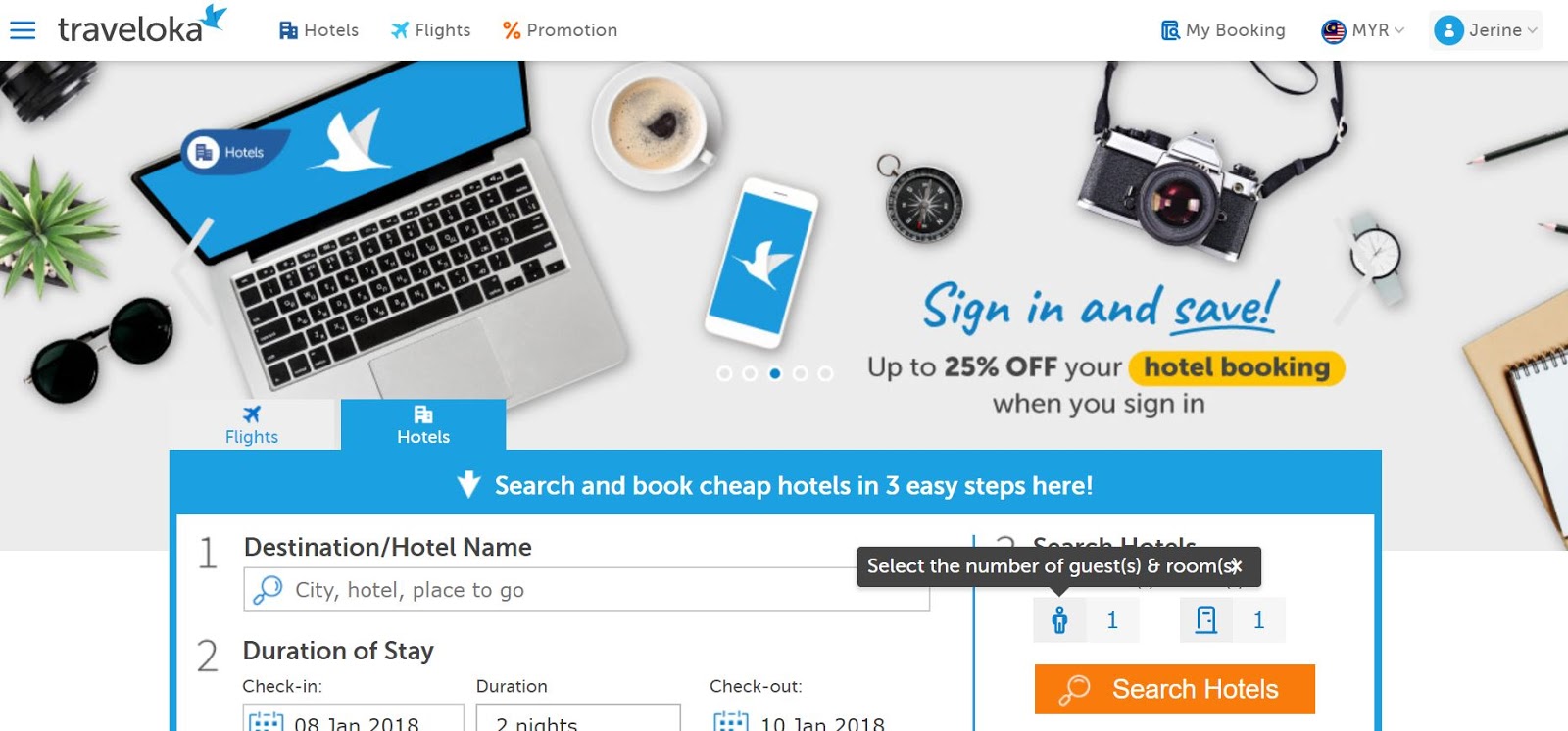This detailed screenshot captures the interface of the travel site "Traveloka." On the left, the recognizable "T-R-A-V-E-L-O-K-A" logo is prominently displayed alongside a small bird graphic. Adjacent to this are sections labeled "Hotels," "Flights," and "Promotions," each accompanied by its respective icon. On the right side, there's a section labeled "My Booking," featuring a flag icon and displaying "M-Y-R." Next to this is a human figure icon with the name "J-E-R-I-N-E" beside it.

Below the header, the screenshot transitions to a photograph showing an individual's workspace. The image includes a laptop open to the Traveloka website, with the recognizable bird logo on the screen. The same webpage is visible on a smartphone beside the laptop. The desktop setup is composed of a cup of coffee, a camera, a pair of sunglasses, and a small potted plant. A prominent blue font on the webpage encourages users to "Sign in and Save," offering up to 25% off hotel bookings for those who sign in. Below this banner, there are fields for inputting information such as destination, hotel name, duration of stay, number of guests, and rooms, alongside a search button to find suitable hotel options. This snapshot of the Traveloka website encapsulates its user-friendly layout and promotional offers.